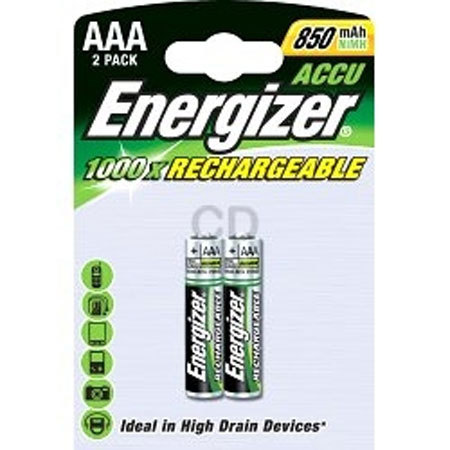This image features a battery pack, specifically an Energizer AAA 2-pack. The package, designed for retail display, includes a hole at the top-center for hanging on a store rack. At the top left corner, the packaging is marked with "AAA 2 Pack." A prominent yellow tab showcases "850 mAh," and directly below it, in green text, it reads "Energizer." Further down, "1000X" and "Rechargeable" are highlighted in bold yellow letters.

The packaging displays two Energizer AAA batteries, each marked with a "C" and a "D." An array of green circular icons runs down the left side, showcasing various high-drain devices like cell phones, headphones, a video game handheld console, a camera, and additional headphones. The phrase "Ideal for high drain devices" is featured prominently, emphasizing the batteries’ suitability for such gadgets. The entire battery section is set against a crisp white background, ensuring all details are easily visible.